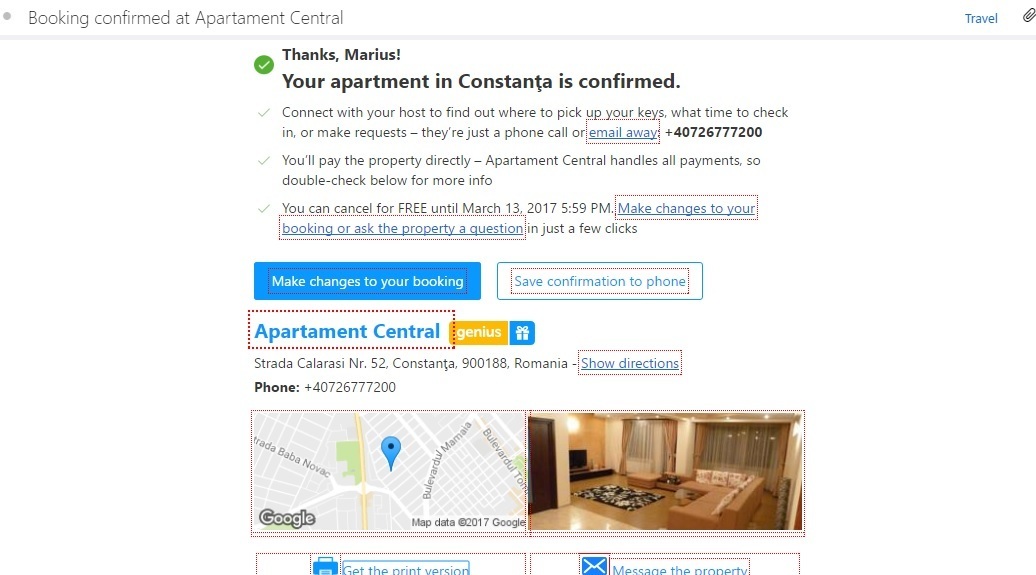This image appears to be a screenshot from a webpage confirming a booking at "Apartment Central." At the very top, it features a bullet point with the text "Booking confirmed at Apartment Central." Directly below, a gray horizontal line spans the width of the section. Toward the far right end of this line, the word "Travel" is highlighted in blue, accompanied by a paperclip icon.

Beneath this header, there is an acknowledgment message that reads, "Thanks Marius!" followed by a green circular icon with a white checkmark. The text "Your apartment in Constanta is confirmed" is prominently displayed next.

Further down, three bullet points provide additional details and suggestions:

- Connect with your host to find out where to pick up your keys, what time to check-in, or to make requests. They are just a phone call or email away, with clickable options for contacting via phone or email.
- Additional instructions or features similar to the first, though not specified.
- Another point of reference offering similar guidance, details not given.

Continuing down the page, there’s a blue rectangular button labeled "Make changes to your booking." Adjacent to it is a visually distinct button that reads "Save confirmation to phone," edged with a red outline within a blue border, making it appear white inside.

Next, the text "Apartment Central" is bordered by a blackish line with a faint pink overlay. Additionally, a yellow label marked "Genius" is visible.

Finally, at the bottom of the page, there are two sections: one displaying a map and the other showing a picture.